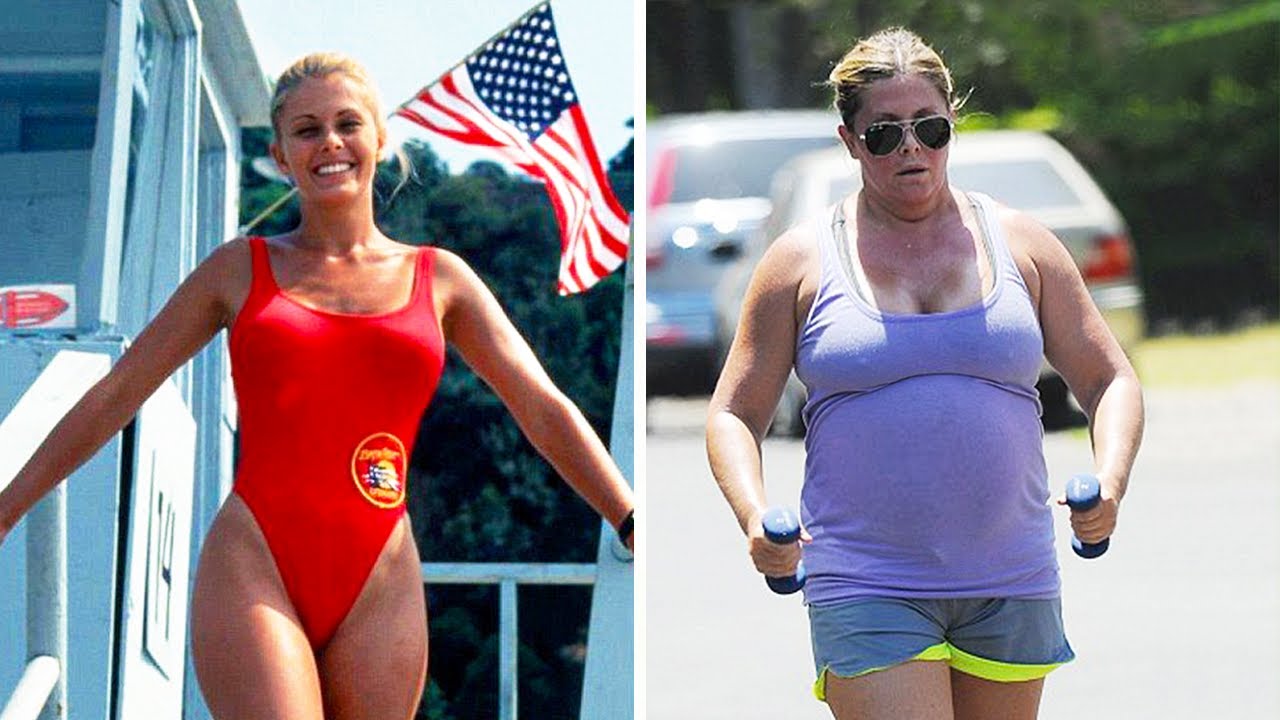The image is a side-by-side composition of two separate photographs featuring two females. On the left, an attractive young blonde woman with a fit physique and well-developed muscles is smiling broadly, showcasing her beautiful white teeth. She is dressed in a red one-piece swimsuit and stands on the steps of a lifeguard station at a beach, with an American flag waving prominently behind her against a bright, sunny backdrop. On the right, a middle-aged, overweight woman is walking down a residential street while exercising. She is wearing sunglasses, a lavender tank top, and grey exercise shorts with yellow accents, and is holding a small dumbbell in each hand. Focused on her workout, she appears determined and serious, contrasting with the joyful demeanor of the younger woman.